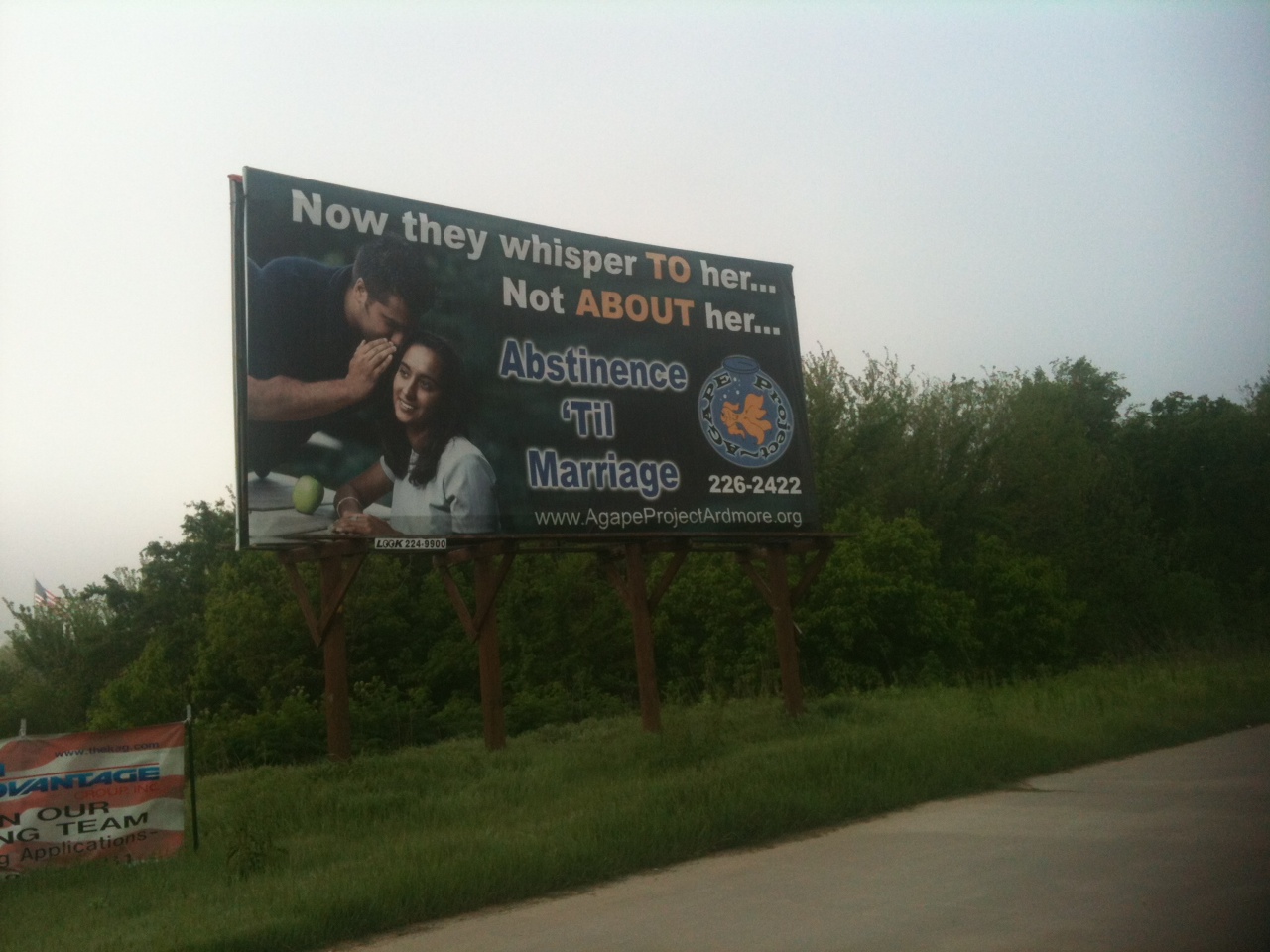This image captures a roadside scene with the backdrop dominated by lush green trees and a cloudy, gray sky. The foreground features a grassy expanse, punctuated by a red and white banner on poles that partially reads "Vantage R Team," though the rest of the text is obscured. The focal point of the image is a large billboard showcasing a young man leaning in and whispering into a young woman's ear. The billboard features bold text, with "Now they whisper to her, not about her" prominently displayed, utilizing a mix of large orange and white lettering for emphasis. Below this message, the billboard advocates for "Abstinence till marriage" and provides a website for more information: www.agateprojectardemore.org.